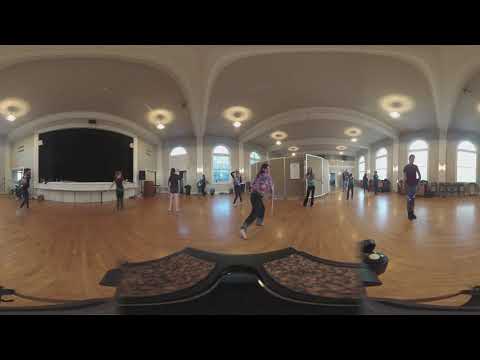The image depicts a distorted panoramic view of a spacious dance studio with a highly polished hardwood floor. The studio is bustling with over ten performers, both males and females, practicing a routine in casual street clothes, rehearsal attire, or exercise costumes such as sweats and tights. The ceiling is a creamy white color, adorned with recessed lighting fixtures resembling the letter "O" with dark centers. To the left, a stage with a black curtain is partially visible. The scene is framed by large arch-shaped glass windows along the walls, allowing ample light into the space. The image appears to be captured with a fisheye lens, as the walls are stretched out and bowed outward with curved lines, creating a visually dynamic effect.